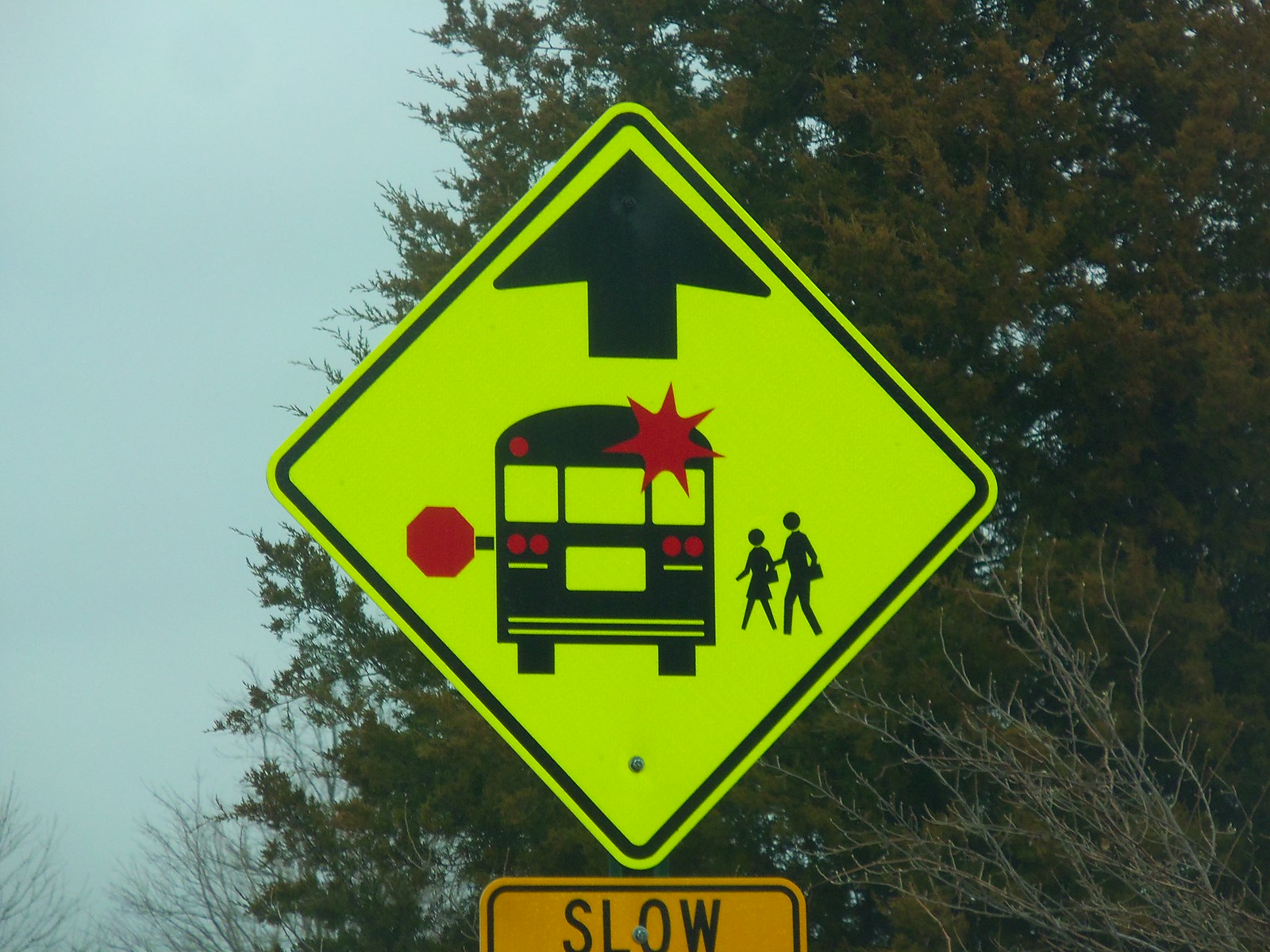This close-up image captures a traffic sign post surrounded by a late fall or early winter backdrop, characterized by leafless trees interspersed with evergreens under a cloudy blue sky. The modern, diamond-shaped, neon yellow-green sign, known as "strong green" by the DMV, features a bold black border and a prominent black arrow pointing upward, indicating an upcoming bus stop. Central to the sign is a black silhouette of a school bus with red highlights, such as a stop sign extending from its side. Adjacent to the bus are two black silhouette children, warning drivers of the nearby bus stop. Below this modern sign, a smaller, old-fashioned yellow sign with partially visible black lettering reads "SLOW." Both signs are affixed to a metal post with noticeable gray screws, emphasizing the caution required in this area.